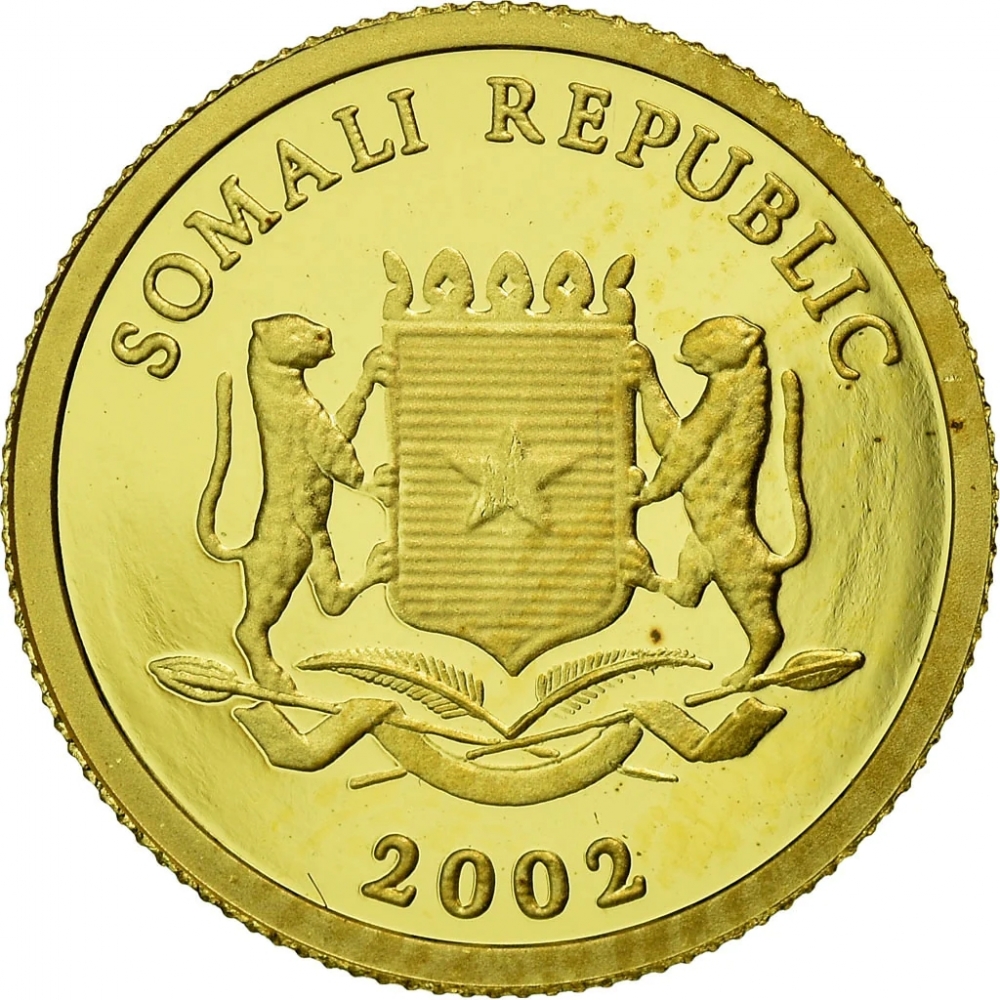The image prominently features a large, textured gold coin with ridges along its rim and a solid band encircling a lighter gold central area. The top of the coin bears the inscription "Somali Republic," while the bottom displays the year "2002." The coin's focal point is a crest held by two cheetah-like or panther-like animals standing on their hind legs. The crest itself has horizontal stripes and a five-pointed star at its center, topped with a crown-like design. Below the crest are two palm leaves intertwined with a ribbon and two spears, on which the animals appear to stand.